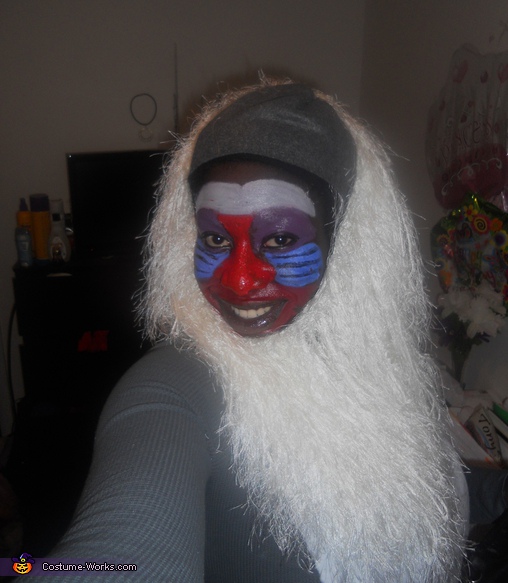The photograph is a selfie of an African-American woman inside a room, dressed up as a character resembling Rafiki from The Lion King. Her face is elaborately painted with a large red nose, blue cheeks, a white forehead, purple around her eyes, and red around her mouth. She is smiling directly at the camera. Covering her entire head is a black wig topped by a white mane that frames her face. She is wearing grey clothes, adding to the essence of a costume. The room she is in has white walls and is somewhat dark, with various items visible such as a table, bottles, and a TV. In the bottom left corner of the image, the website name "costume-works.com" is written.